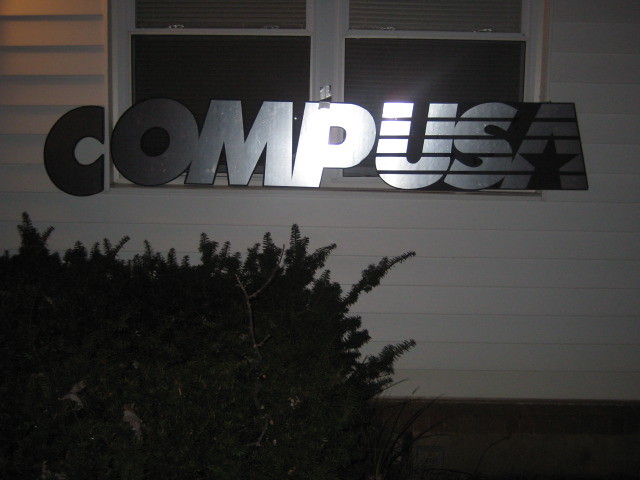In this black and white nighttime photograph, the side of a white building, likely a home, dominates the scene. The building features white siding, which could either be vinyl or wooden boards. At the center of the image, two windows sit side by side, framed by white borders, with blinds visible through the glass. A large silver sign, emblazoned with "COMPUSA," stretches horizontally between the two windows. The letters "C," "O," "M," "P," "U," "S," and "A" are prominently displayed, with the "USA" distinguished by bold black streaks across the letters. Notably, a light shines just above the "P," casting a glow that highlights the central portion of the sign. To the bottom left of the building, a substantial shrub appears, almost black due to the image’s dark tones, with its lush and thick foliage pressing against the house. The ground in the bottom right corner also appears black, contributing to the image's overall dim and nocturnal ambiance. A small segment of the concrete foundation is visible at the bottom of the building, adding to the detailed composition of the photograph.